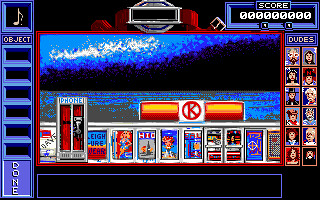This landscape-mode screenshot from a vintage-style video game, characterized by its simplistic, pixelated graphics, captures a busy and somewhat cryptic scene. The background, predominantly black and blue, prominently features what appears to be water and a large wave near the top of the screen, suggesting a potential theme centered around surfing or ocean activities. In the upper right corner, a scoreboard displays a score of zero. 

On the right side of the image, arranged in two columns of six rows, are computer-generated illustrations titled "dudes," depicting head-and-shoulder portraits of twelve different individuals. The upper left corner of the screen features an object area with a musical note icon and the word "done" at the bottom. 

The bottom section of the screen includes several rectangular icons; one notably taller than the others resembles a red phone booth. Despite the clutter of various icons and images, specific details remain difficult to discern. A prominent "Circle K" in the center and the overall aesthetic evoke a nostalgic, old-school video game atmosphere.